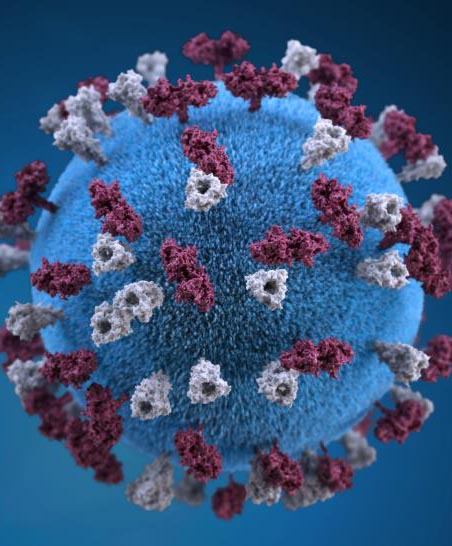This image is a detailed computer-rendered illustration of a virus, set against a dark blue background. A large, fuzzy blue orb occupies the center of the image, featuring numerous short, spiky strands on its surface. Sprouting evenly across the entire surface of the blue sphere are tiny structures resembling trees, distinguished by their crimson red and off-white colors. Each of these trees has a hole at the top, enhancing the biological, almost microbial, aesthetic of the depiction. The focus is sharply centered on the front of the orb, making its detailed structures prominent, while the edges and background of the orb fade out of focus, emphasizing the central features. This abstract and highly detailed portrayal evokes the microscopic appearance of a virus, possibly even a coronavirus, given its distinct color scheme and spiky projections.